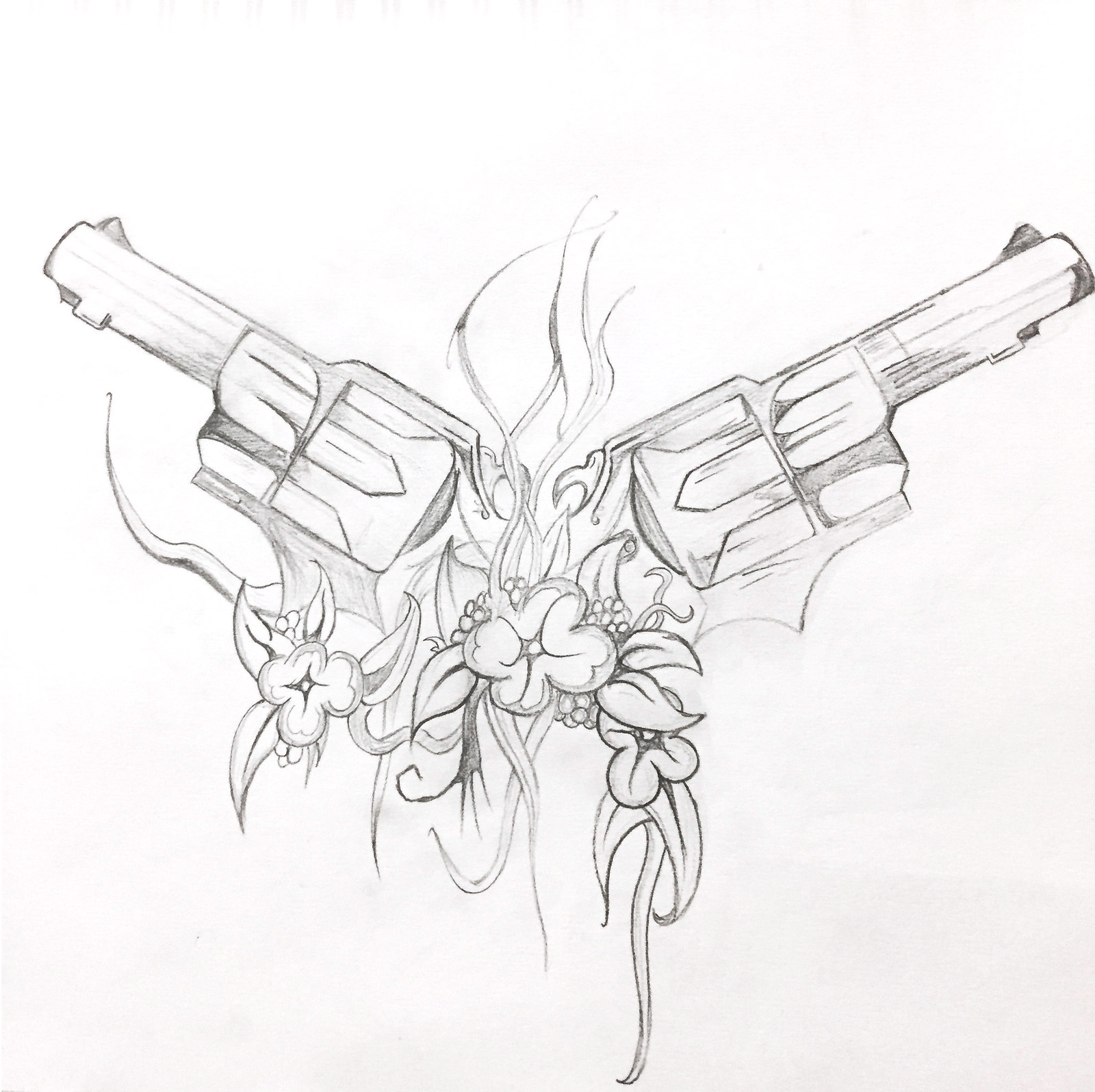This black-and-white sketch presents a detailed, symmetrical composition featuring two pistols oriented outward—one facing left, the other right. The visible parts of the guns are primarily the barrels and cocking mechanisms, while their handles remain hidden. Between the guns, vibrant with detail, are three four-petaled flowers, forming a central focus. The flowers are surrounded by an intricate array of elements: clusters of small circular shapes, long pointed leaves, and what could be interpreted as longhorn steer antlers or flames, adding an eclectic, almost bouquet-like arrangement. The combination of floral and firearm elements creates a striking contrast, suggesting that this sketch might be intended as a potential tattoo design.